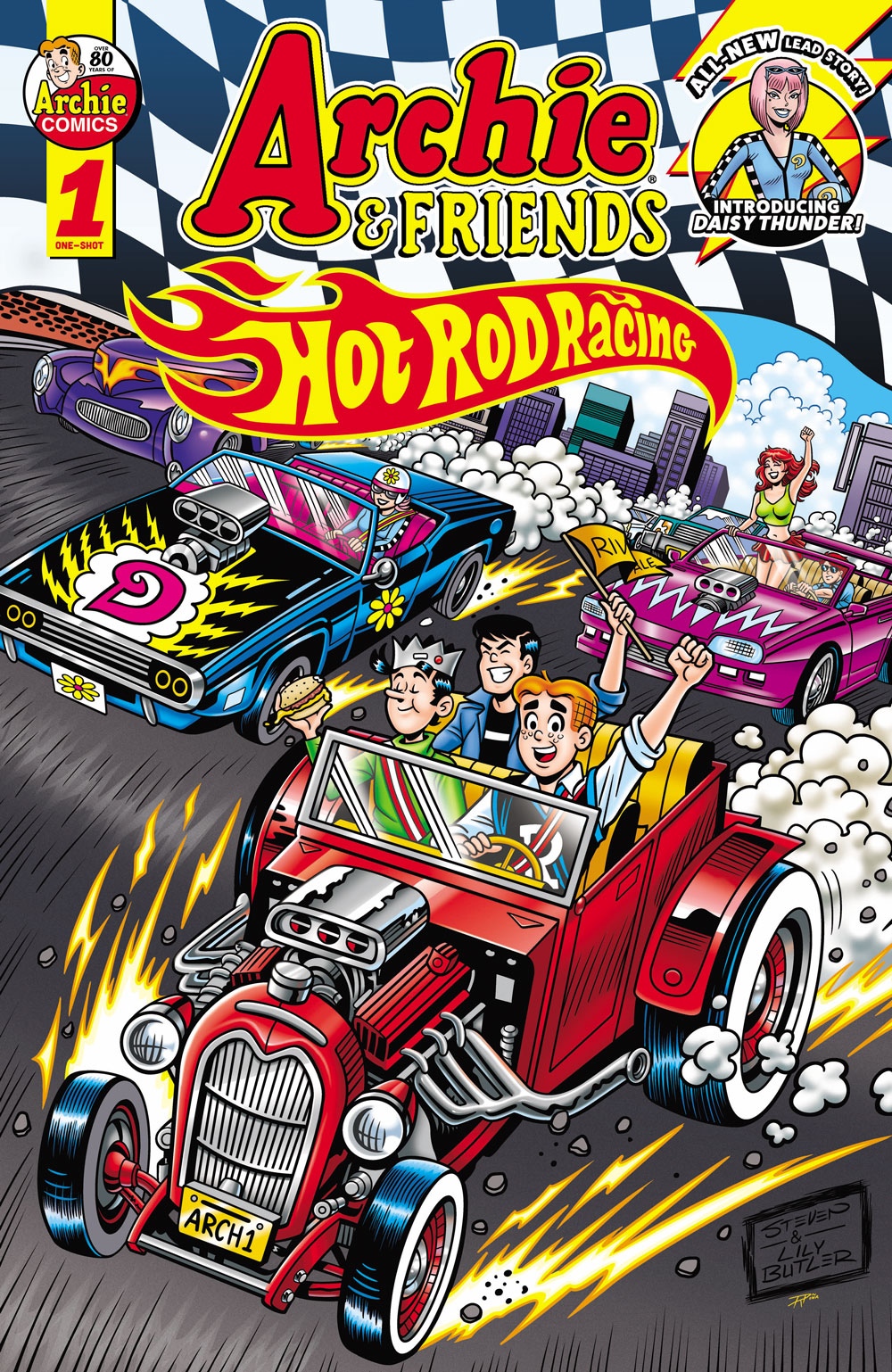The image is a vibrant, action-packed cover of an Archie and Friends comic titled "Hot Rod Racing," evidently styled after Hot Wheels. Dominating the top, the title "Archie and Friends" shares space with the "Hot Rod Racing" subtitle and the iconic Hot Wheels logo. The top right corner announces an all-new lead story by introducing Daisy Thunder, a charismatic character depicted with a hot pink bob haircut, cat-eye sunglasses pushed up on her forehead, thick makeup, and a devious smile. She dons a blue racing suit adorned with a yellow 'D' over her right breast.

A circular emblem in the top left corner celebrates "over 80 years of Archie comics" with a red '1' labeled "one shot" beneath it. Below this, Archie and his friends are engaged in an enthusiastic road race. Archie, with his signature red hair and freckles, is in the driver’s seat of an old-fashioned red convertible, his right hand on the steering wheel and his left fist raised in the air. Next to him, Jughead, wearing his crown hat and a green turtleneck, holds a hamburger. Reggie, seated in the back, has a huge smile, eyes shut, and waves a Riverdale pennant.

Behind them, Daisy Thunder charges ahead in a distinct blue convertible featuring a cloud design with lightning bolts and a large pink 'D' on the hood. She drives with both hands on the wheel, wearing a white helmet with a daisy and blue jumpsuit, in a car whose hot pink seats stand out. To her right, another car—a pink convertible—has a young man with red hair at the wheel and a woman standing beside him. With long red hair flowing, she grips the front windshield with her right hand and raises her left fist joyously. The background teems with city skyscrapers, cauldrons of motion lines, flames, and smoke emanating from the vehicles, embodying the high-octane energy and spirit of competition in this engaging comic cover.